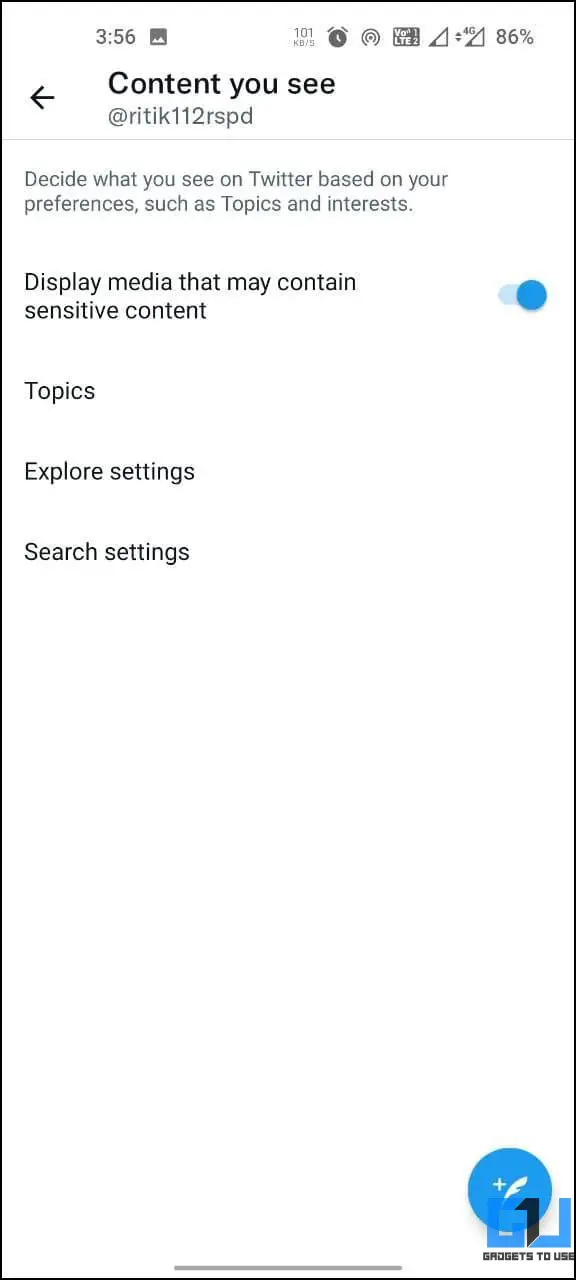This mobile screenshot, vertically oriented and bordered by a thin black line, appears to display a settings page from the Twitter app. The layout consists of a white header and main screen, creating a clean and minimalistic aesthetic. 

At the very top left corner, within an indented section, the number "356" is visible. To the right, there are six small icons, indicating various functions, with the battery level at 86%. 

The header prominently features the title "Content UC" accompanied by a left-pointing arrow, suggesting a navigation option. Directly underneath, the text "@RITIK 112 RSPD" is displayed, possibly referring to the user or account settings.

A thin gray horizontal line separates the header from the main content. The leading text in the main content reads, "Decide what you see on Twitter based on your preferences such as topics and interests." This is followed by the phrase, "Display media that may contain sensitive content," next to which is a small blue toggle switch set to the 'on' position.

Further down, three options are listed: "Topics," "Explore settings," and "Search settings," inviting the user to further customize their experience. The majority of the page remains blank, emphasizing its simplicity.

In the lower right corner, there is a distinctive blue logo featuring a circle with a plus sign, a feather, and the initials "GU" in a stylized font, hinting at a related feature or branding. The image is concluded with a thin gray line at the bottom center.